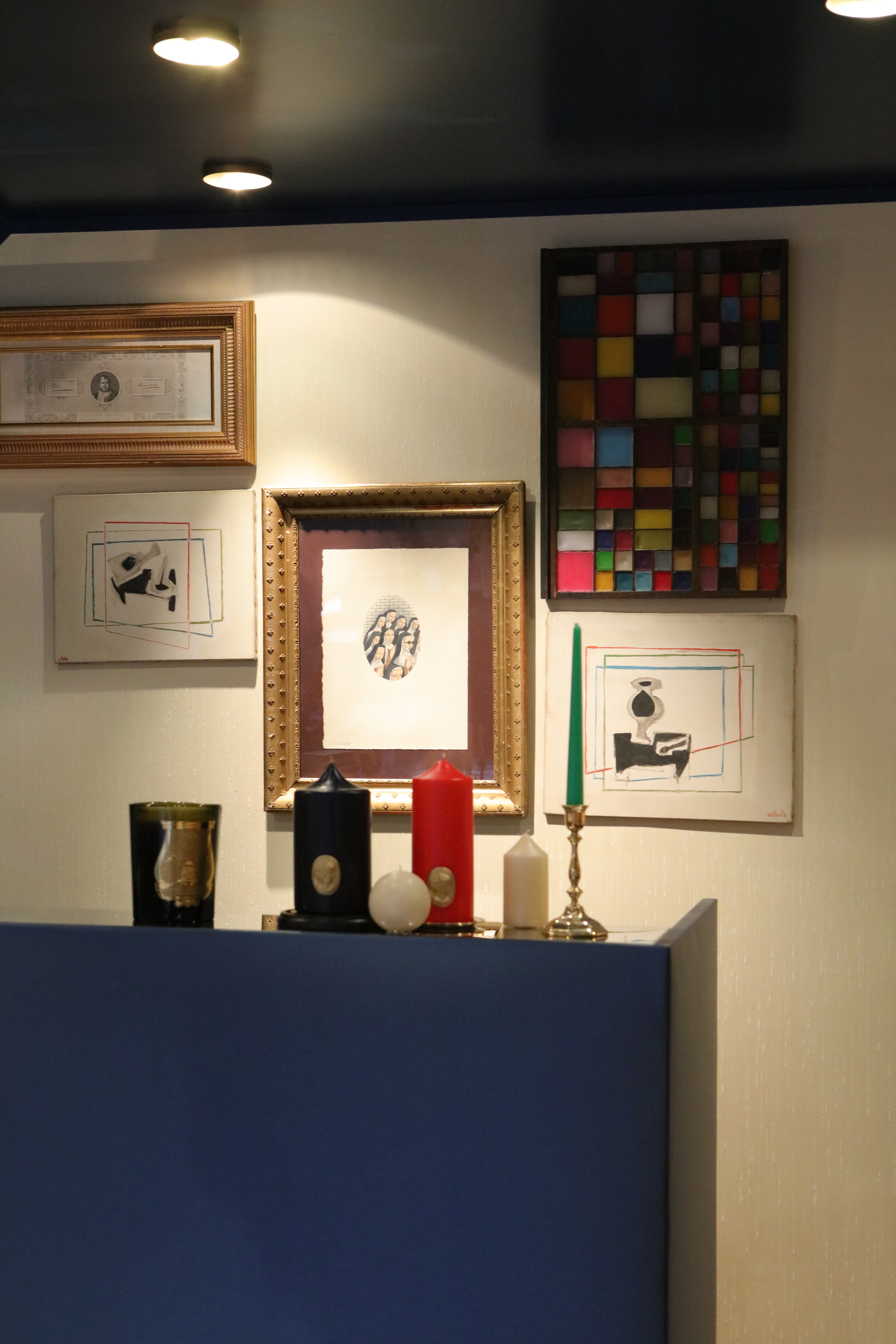The photograph showcases the interior of a business setting with a tall blue counter dominating the foreground. Atop the counter sits an array of decorative candles: a black candle and a red candle, both on a tray, flanked by a smaller spherical white candle. A larger white candle resides close by on a slightly lower surface, next to a gold candle holder cradling a tall green candle. Additionally, there's a chrome and black cup present on the counter. The background features a stark white wall adorned with various artworks and frames. A detailed montage, comprised of multicolored squares, occupies the top right corner, beneath which lies a barely distinguishable drawing. Moving left, a picture with a white and red backdrop framed in gold captures attention, adjacent to another indecipherable plaque and a drawing comprising various shapes in the top left. The black ceiling overhead houses lighting that illuminates the scene, with an encased frame displaying what appears to be military medals adding a touch of distinction to the decor.